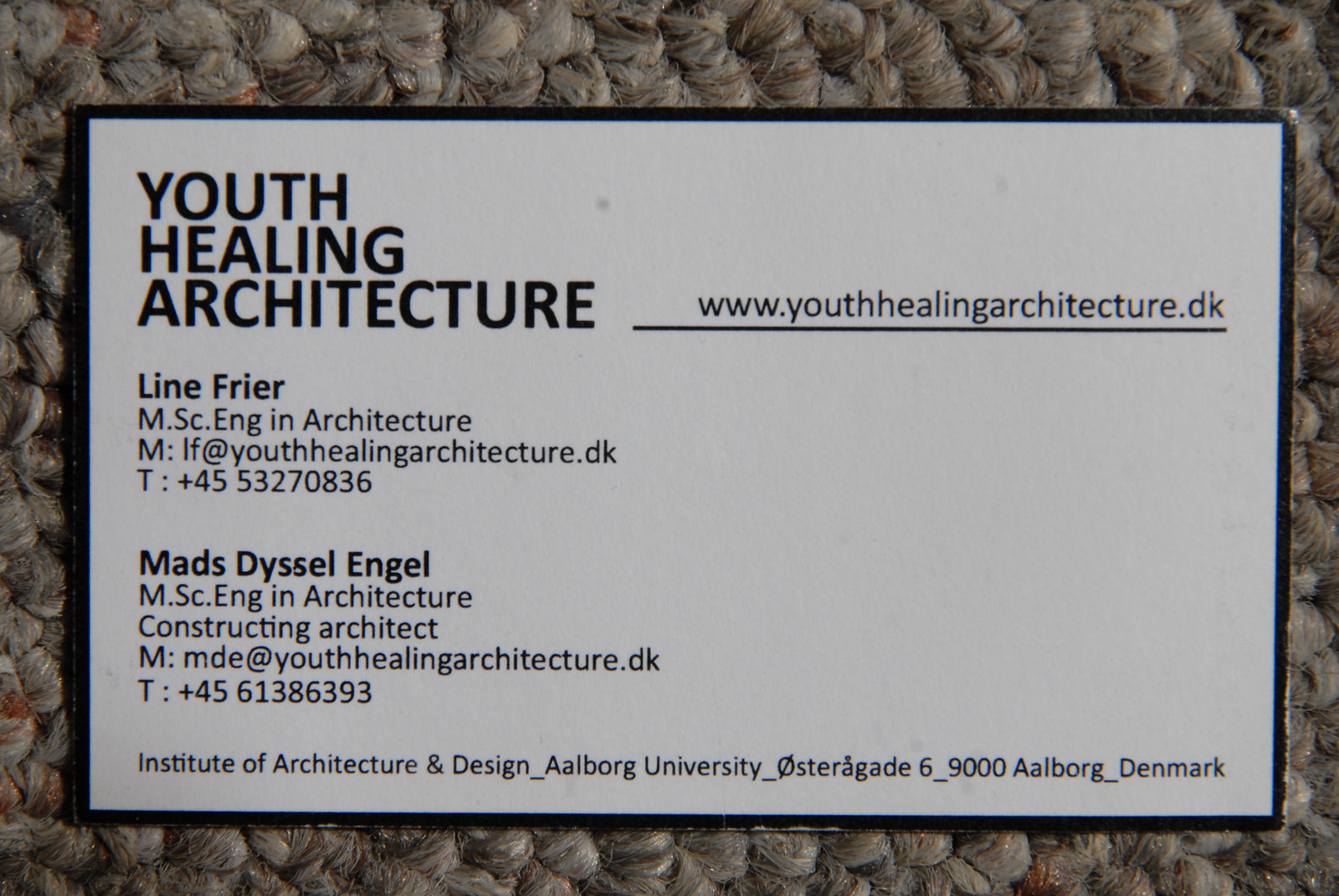This is a detailed close-up photograph of a business card resting on what appears to be a textured fabric or carpet background. The business card features a predominantly white background with a flat black border. The text on the card is primarily in black. 

In the top left corner, the card displays the name "Youth Healing Architecture" along with the website "www.youthhealingarchitecture.dk." Directly beneath this, the card lists two names: "Line Friar, MSc. Eng. in Architecture," with a contact email "mif@youthhealingarchitecture.dk," followed by a phone number "+45 61386393." Below Line Friar's details, it mentions another individual, "Mads Diesel Engel, MSc. Eng. in Architecture, Constructing Architect," with the email "mmde@youthhealingarchitecture.dk" and the phone number "+45 61386393."

On the right side of the card, an email address is provided. At the bottom of the business card, it states "Institute of Design and Architecture," and provides further details: "Aalborg University, Østerågade 6, 9000 Aalborg, Denmark." This comprehensive information is arranged in a neat and orderly format, allowing for clear and easy reading.